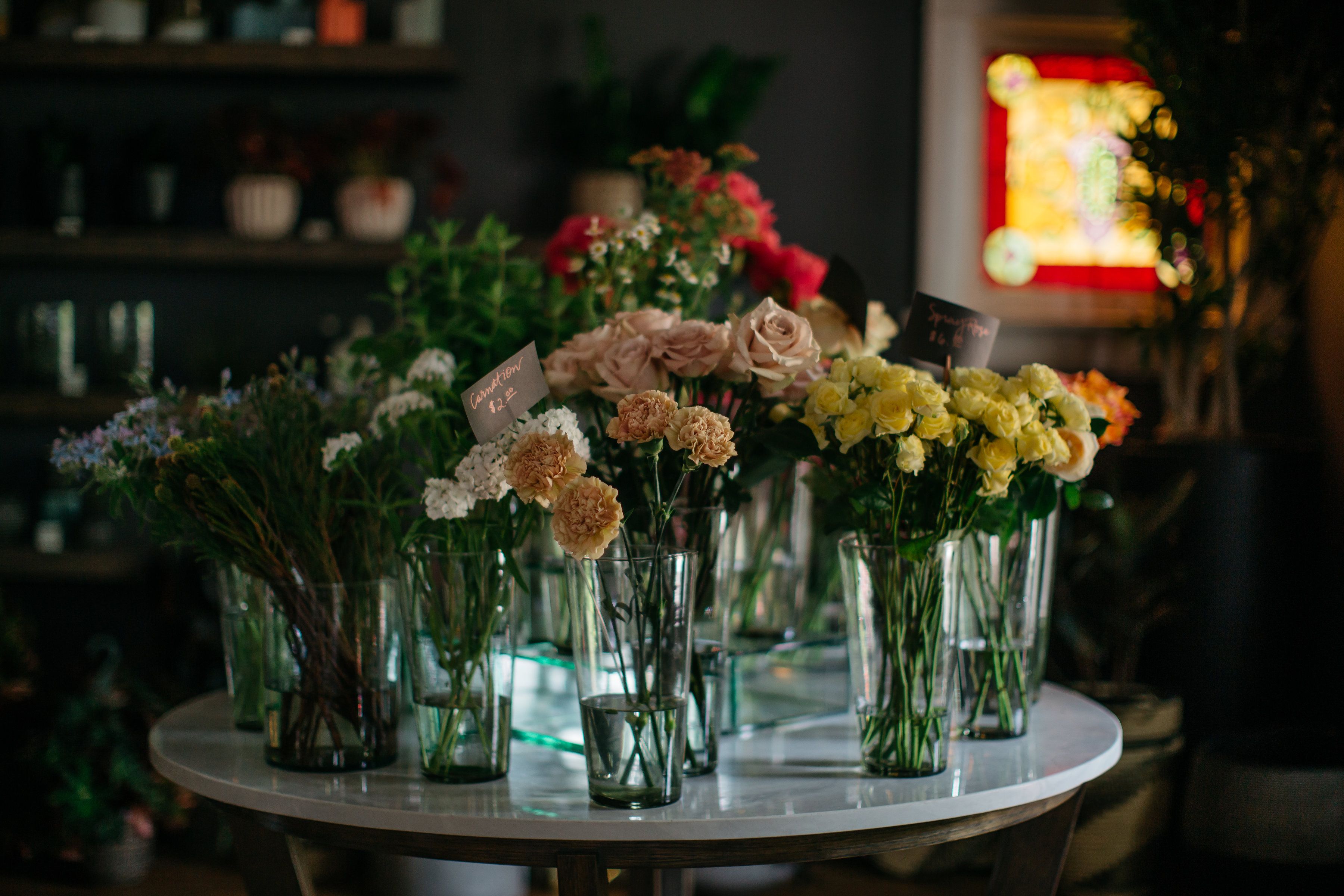The image captures an indoor scene in low light, showcasing a small, round table with a white marble top and a visible metal base. On the table are several clear glass vases reminiscent of large drinking glasses, each holding long-stemmed flowers. The most prominent flowers are yellow and white chrysanthemums, with two vases containing yellow chrysanthemums and another two with white ones. There is a single vase featuring an orange chrysanthemum and another with pink roses. Additionally, one vase holds blue violets. The vases are arranged to highlight the various colors, creating a vibrant display despite the subdued lighting. In the blurred background, one can see a large bouquet of red roses. The backdrop also includes a stained glass window on the right, casting red and yellow light into the room, and shelves with additional flower pots on the left. Overall, the combination of different colored flowers and the elegant marble table creates a visually striking composition.